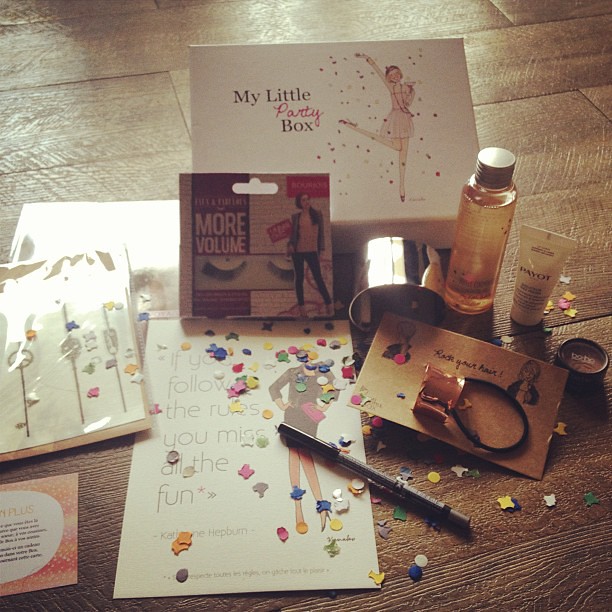This is a detailed photo of various party favors laid out on a wooden floor. The backdrop features a white box labeled "My Little Party Box," adorned with an image of a woman standing on one foot, dressed in heels, and tossing glitter and confetti into the air. The contents of the box are captivating and diverse, including jewelry such as bracelets, a white card that reads "If you follow the rules, you miss all the fun," and a variety of beauty products. These beauty items encompass lip gloss, lotion, perfume branded with "rack your hair," and a hair tie. Additionally, there's a noteworthy inclusion of a pin and a pair of fake eyelashes. Scattered around these items are confetti pieces shaped like stars and circles, enhancing the festive atmosphere.